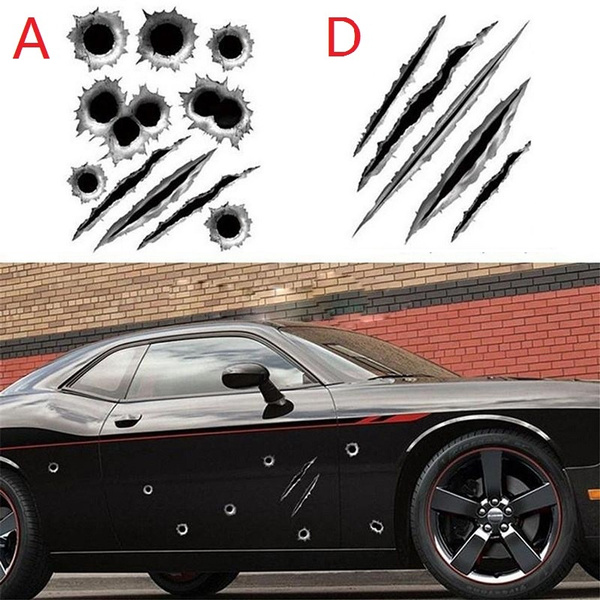The image is a square, four inches by four inches, divided into two sections. The top half features a plain white background showcasing decal samples. On the left, there is the letter 'A' in bold red print, with round black bullet hole decals outlined in silver-gray around it. To the right, there's the letter 'D' in bold red, accompanied by slash mark decals oriented towards the upper right corner.

The bottom half of the image displays a black, two-door sports car, reminiscent of a Dodge Charger, parked in front of a red and brown brick wall. The car's right side is adorned with multiple black bullet hole decals and two large slash marks on the door. The car also features dark metal rims with a five-spoke design and a small red horizontal stripe along the side.

The top section of the image highlights the individual decals, marked as 'A' for bullet holes and 'D' for slashes, indicating how they appear when applied to the car, as demonstrated in the lower section of the image.